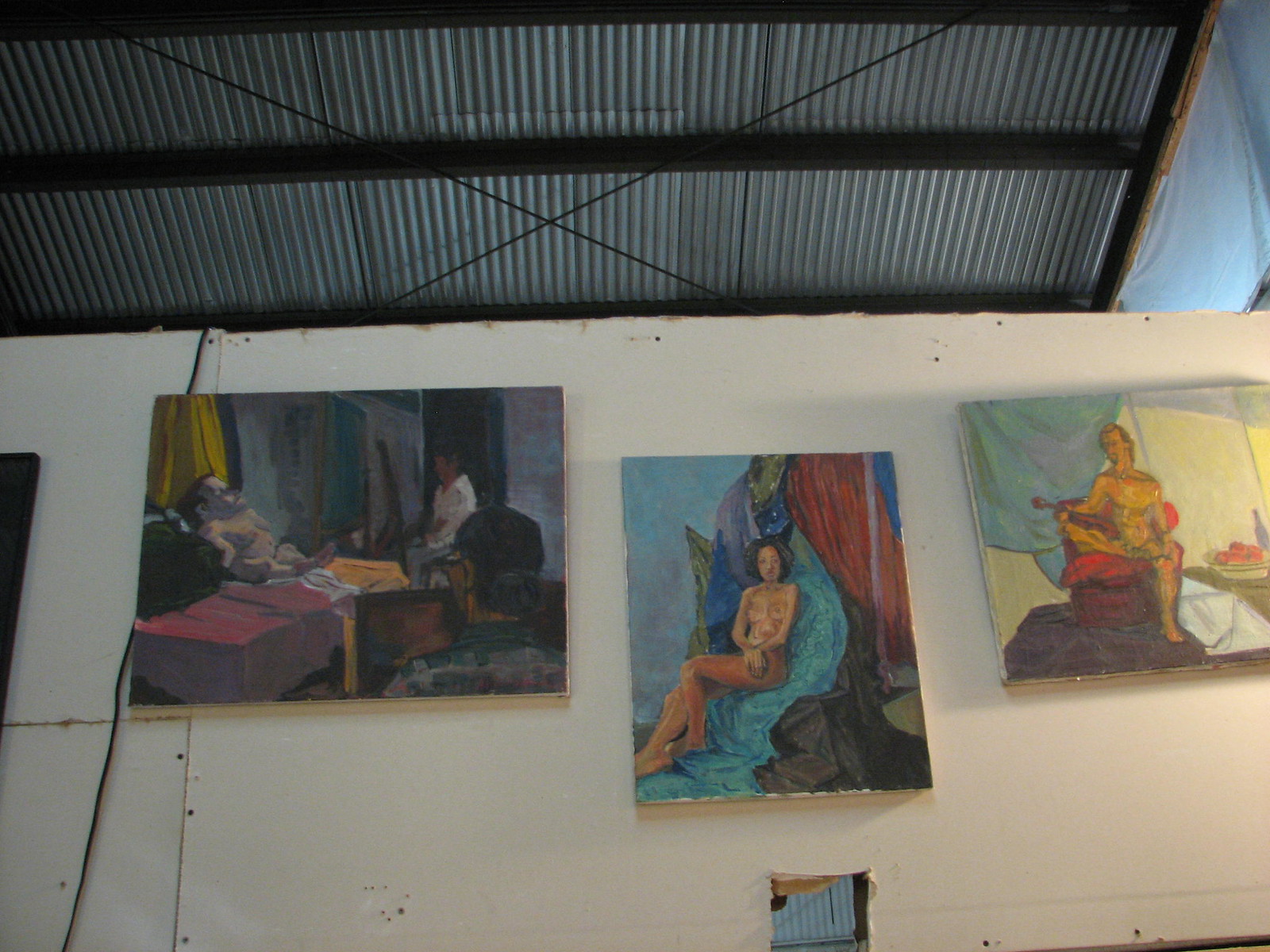This real-life photograph captures an upward-angled view of a tall white wall adorned with three distinct paintings. The white wall occupies approximately 60% of the image, starting from the bottom, with a visible ceiling featuring silver rails and black beams above.

Starting from the left, the first painting illustrates a scene with a man, semi-reclined on a bed, interacting with another person seated in a chair. Clothes are scattered around, and a green rug lies on the ground, all rendered in a style suggestive of watercolors. 

The middle painting features a topless woman sitting on a blue chair, her arms crossed in front of her. She is set against a backdrop of various fabrics in hues of red, green, and dark gray.

The rightmost painting depicts a nude man seated on a red chair next to a table holding a bowl of apples and a bottle. 

Positioned centrally on the lower part of the wall is a small, approximately six-inch square hole. Additionally, there is a white cord running vertically next to the left painting. The paintings exude an abstract, possibly Caribbean or South American influence, adding vibrant, multicultural elements to the stark white background.